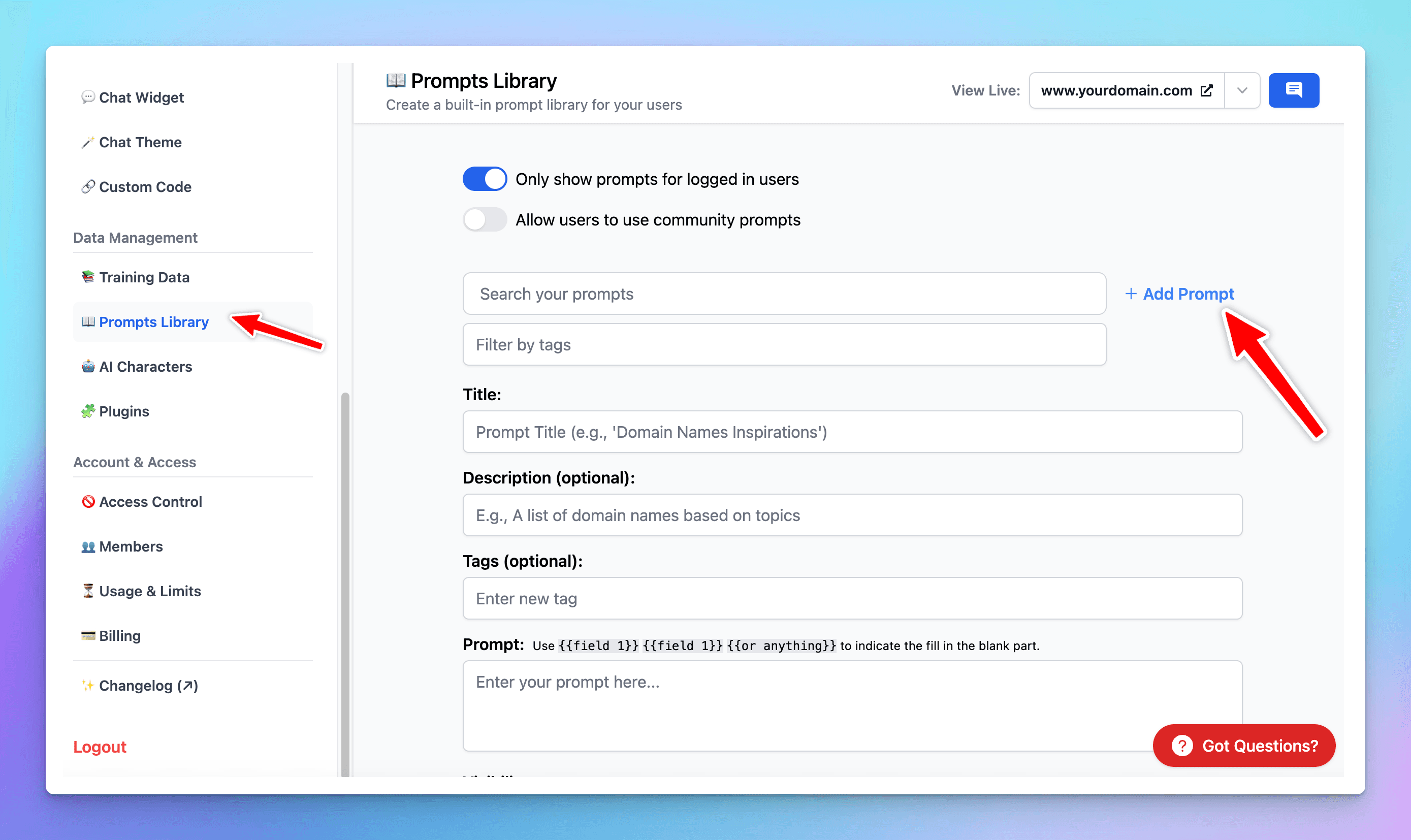This detailed caption offers a comprehensive overview of the image described:

---
The image is a screenshot of a software application interface, specifically a window titled "Prompts Library." The window has been resized and does not occupy the full screen, revealing a background with a blue and purple gradient effect. Within the "Prompts Library" window, a vertical sidebar on the left displays various menu options organized into different sections.

The first section lists:
- Chat Widget
- Chat Theme
- Custom Code

The second section, labeled "Data Management," includes:
- Training Data
- Prompts Library
- All Characters
- Plugins

The third section, titled "Account and Access," features:
- Access Control
- Members
- Usage and Links
- Billing
- Change Log

At the bottom of the sidebar, there's an option to "Log out" highlighted in red text.

The main interface of the window centers on the "Prompts Library," with a header that reads, "Create a built-in prompt library for your users." Directly below, two settings are displayed: "Only show prompts for logged-in users," which is toggled on, and "Allow users to use community prompts." Several input fields for configuration are visible but remain empty. These fields include Search, Tag, Title, Description, Tags, and Prompts, offering spaces for users to fill in necessary details for their prompt library.

This meticulous description provides clarity on both the layout and functionality of the "Prompts Library" interface as seen in the screenshot.

---

This caption aims to be as detailed and descriptive as possible, ensuring that all elements of the image are clearly communicated.